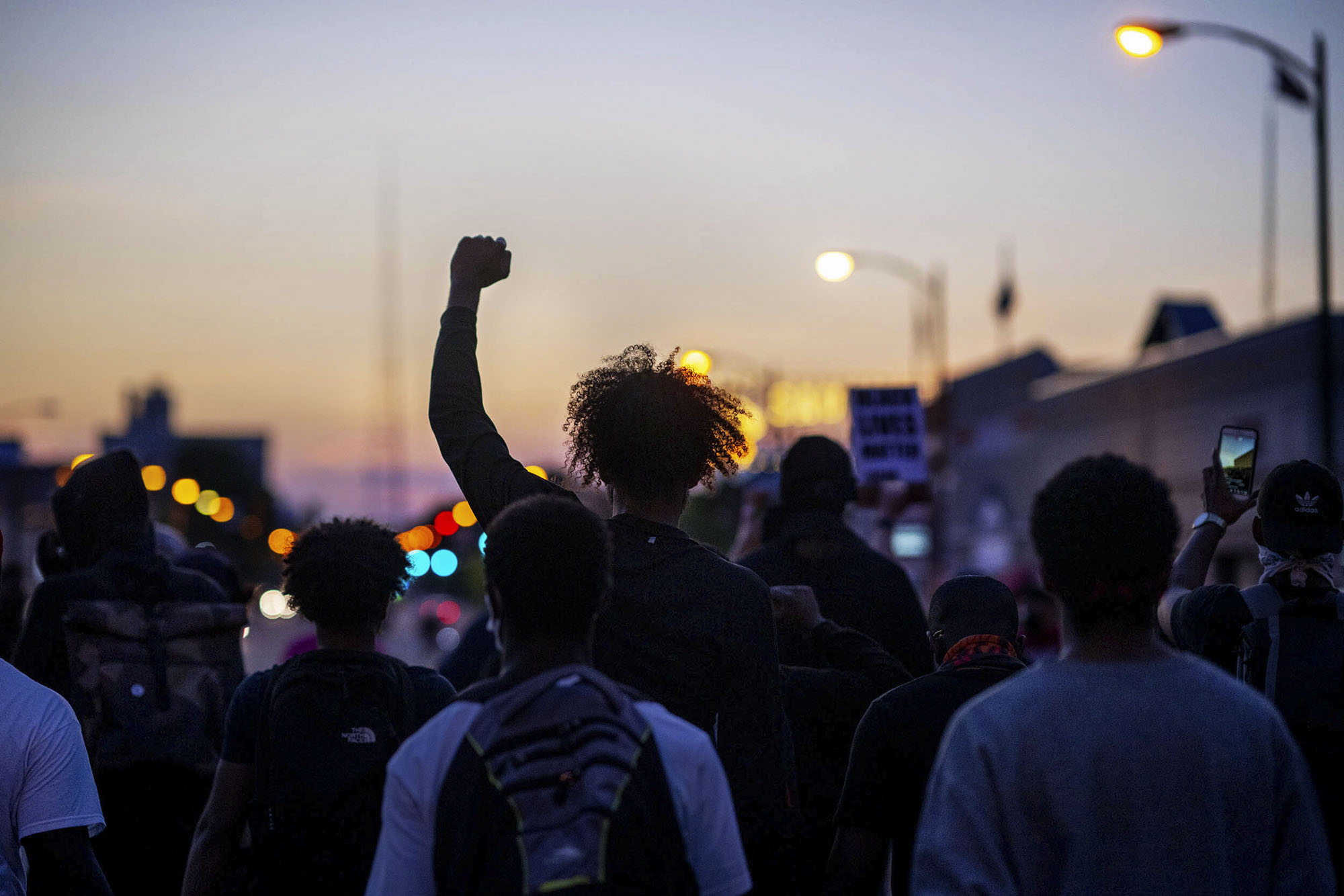This photograph captures a vibrant protest march taking place at dusk. The sky transitions from a grayish hue at the top to a yellowish-pinkish tone near the horizon, tinged with orange and purple as the sun sets. In the foreground, a young man with his left fist thrust into the air stands prominently among a crowd of predominantly young African Americans, many of whom have their backs to the camera. One individual wearing a white long-sleeved shirt and a gray and black backpack leads the march, while another person on the far right is recording the scene with a backlit smartphone. Although the sign that someone holds up is too blurred to read, it emphasizes the rallying spirit of the gathering. The image includes blurred streetlights and colorful orbs of light, adding to its dynamic atmosphere. To the right, a small gray building is visible, flanked by two streetlights, and a radio tower can be faintly seen in the distance. The protesters, mostly dressed in dark clothing, march down a street adorned with out-of-focus lights and partially visible signs, creating a layered, almost surreal urban tapestry against the dimming sky.